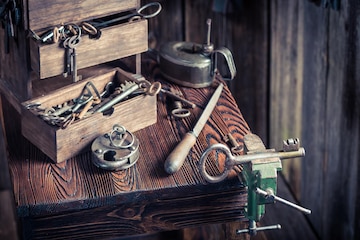In a cluttered indoor shed, a wooden work table showcases various odds and ends. The table, crafted from medium brown wood with a visible grain, is partly occupied by a slender, pale wooden drawer box on the left side. This drawer box has compartments overflowing with numerous skeleton keys, reminiscent of old-fashioned locks. One of its drawers is pulled out and rests on the tabletop, revealing an assortment of metal objects and more keys. In front of the box sits a silver lock with a key inserted.

On the table’s right side lies a sharp tool with a wooden handle, likely a knife or a metal-file, and nearby is a small silver object. Dominating the lower right corner is a green vise grip with silver handles, affixed to the table's edge, holding one of the larger, antique-style keys with a circular bow and basic teeth design. The wooden slats on the shed walls form the background, adding to the rustic, utilitarian ambiance of this workspace.